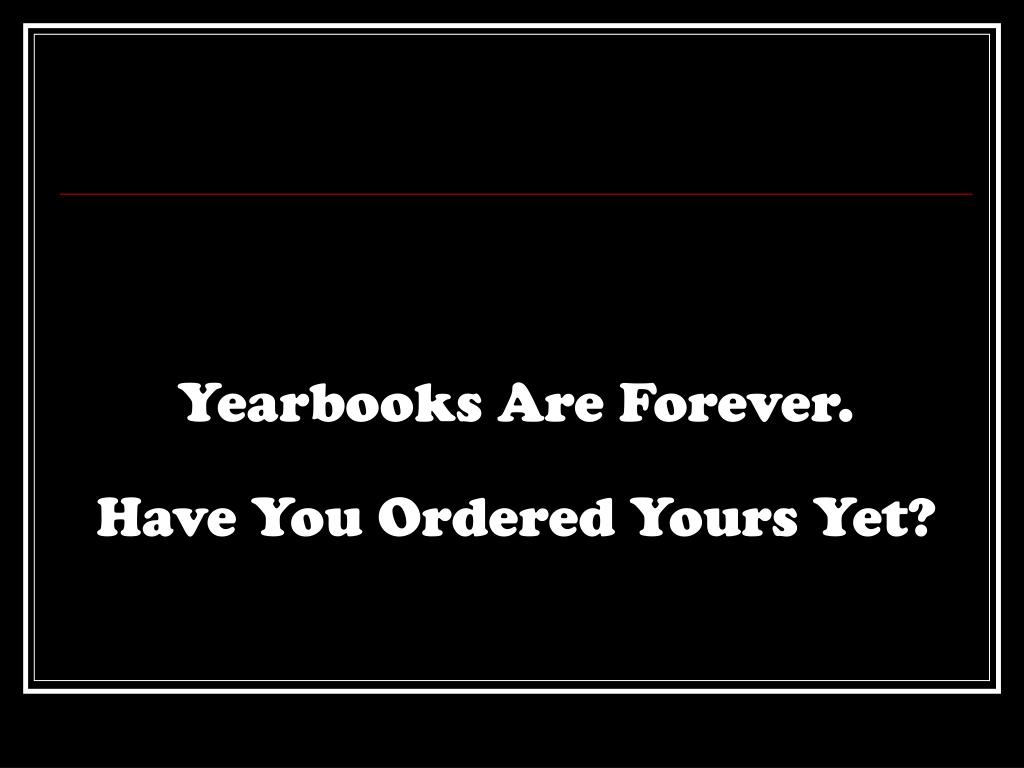The image is predominantly black, featuring a sequence of borders and minimal text. It starts with a large black background, which has a thick white border inset within it. Inside the thick white border, there is a smaller, thinner white border. The inner section, also black, contains a thin horizontal red line placed about a quarter of the way down from the top. Below the red line, closer to the center of the image, is the text in white Cooper font that reads, "Yearbooks are forever. Have you ordered yours yet?" The letters are capitalized at the beginning of each word. There are no additional images or text elements in the design, maintaining a simple yet striking visual presentation.